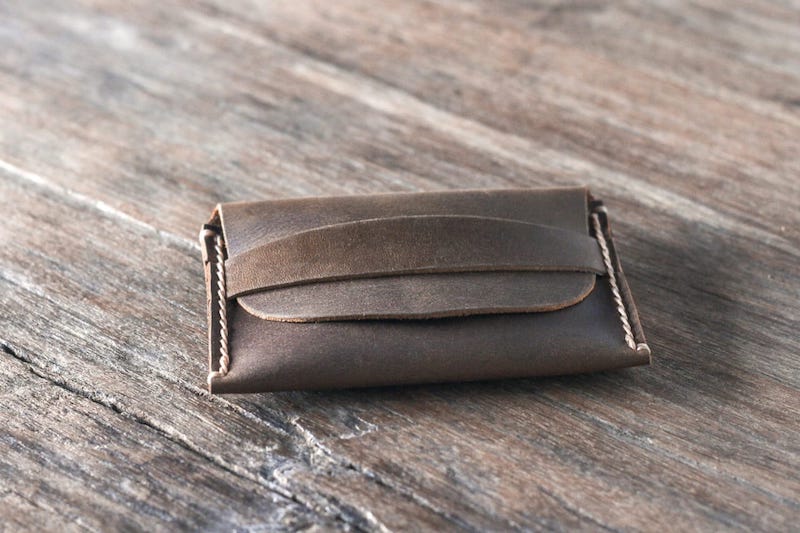This photograph captures a detailed image of a hand-stitched leather case, most likely designed for holding glasses but potentially suitable for a small electronic device. The case is expertly crafted from light brown leather, featuring thick white braiding-style stitching along each side that secures its structure. It has an envelope-style design, bulging in the middle with tapered sides, and includes a sewn-on strap to secure the closing flap. The item, centered in the close-up shot, is laid out on a weathered brown wooden surface that displays noticeable scratches, contrasting subtly with the darker brown shade of the leather. The photograph emphasizes the artisanal quality and intricate details of the stitching, highlighting the craftsmanship of this elegant, multifunctional leather case.